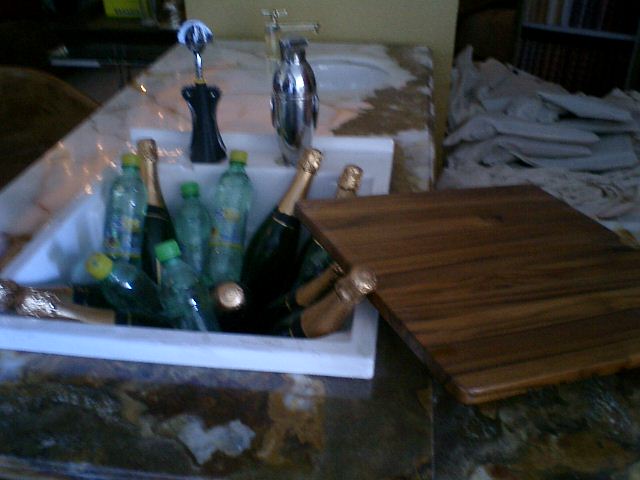The image depicts a scene featuring an ivory white marble countertop with intricate gold and brown patterns. There are two sinks embedded in the countertop: one is a deep, rectangular sink and the other is a round sink with a visible faucet. The rectangular sink is filled with various bottles, including unopened champagne or wine bottles with dark green hues, clear green bottles with caps, and turquoise plastic water bottles. Additionally, there is a wooden mahogany cover, likely a cabinet cover, discarded next to the sink. In the background, a bottle opener with a black bottom and a silver top is visible, along with what appears to be a silver cocktail shaker. The floor is cluttered with white papers strewn across it. The overall image is somewhat unclear, reminiscent of either a blurry photograph or a painting, which adds an element of ambiguity to the detailed kitchen or bathroom setting.